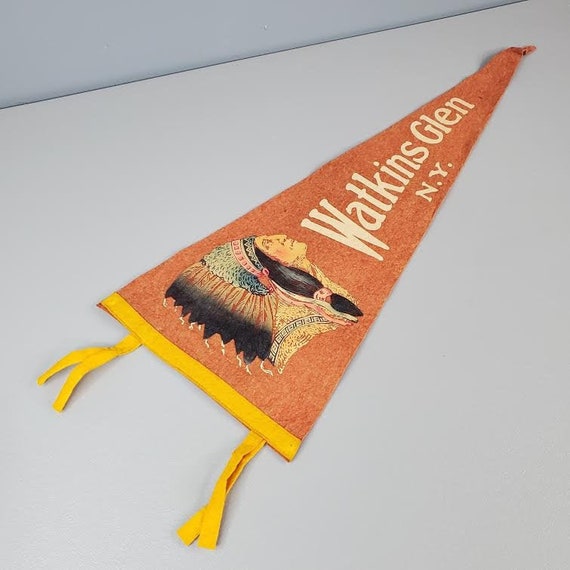This image features a close-up of a detailed, vintage triangular pennant flag, prominently displayed on a light gray wall. The pennant itself is an orangish-brown, with its wide end featuring a goldish-yellow band adorned with two matching tassels. This colorful accent is positioned diagonally from the bottom left to the top right. The pennant, made of felt, has a slightly crumpled tip and is framed against a darker gray ceiling.

Central to the pennant's design is the striking image of a Native American chief, depicted in profile with an elaborate headdress and long black hair, looking to the right. Accompanying this vivid illustration, the text "Watkins Glen, New York" is emblazoned vertically in white, following the pennant’s length. The background and photograph's modern quality highlight the timeless charm of this classic memorabilia.